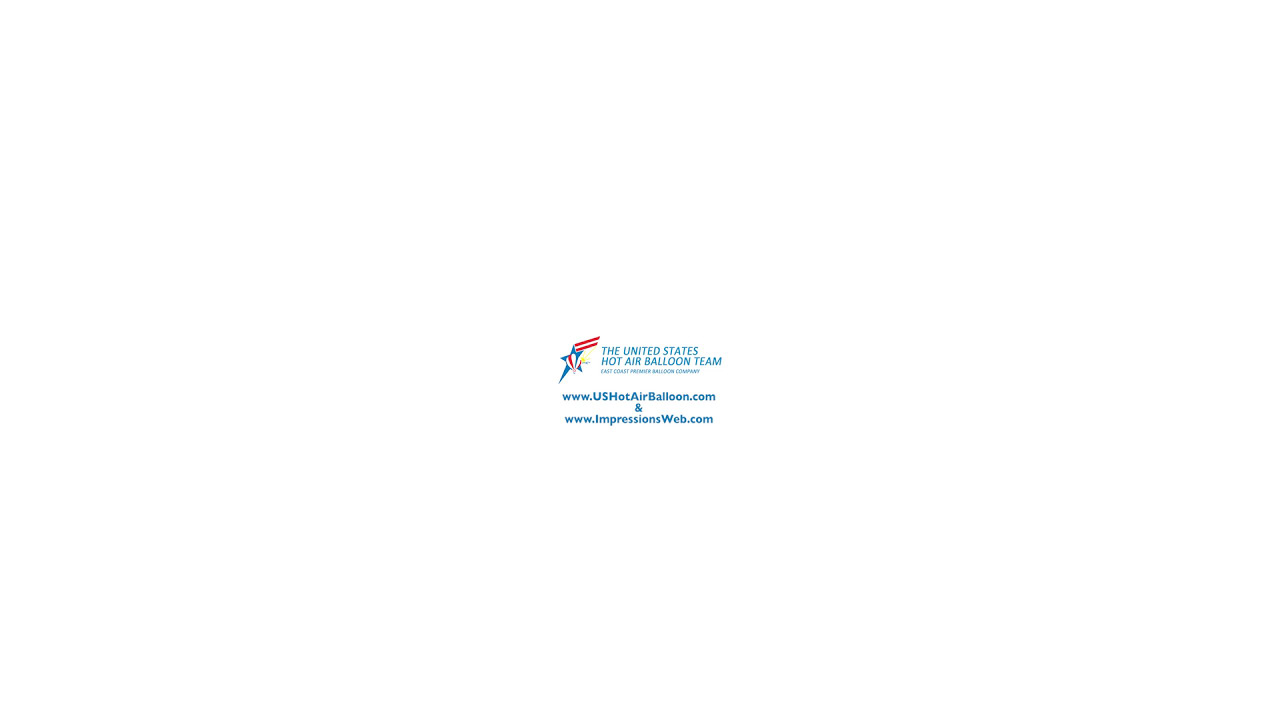The image features a white background with a central graphic element. In the center, there's a logo consisting of a hot air balloon adorned with red, white, and blue stripes, positioned in front of a blue star with red stripes at the top. To the right of the logo, bold blue italic text reads "UNITED STATES HOT AIR BALLOON TEAM." Directly below this is smaller text that may refer to the East Coast Hot Air Balloon Company, though it's less readable. Further down, in bold blue text, are two website addresses: www.ushotairballoon.com and www.impressionsweb.com. The entire design is clean and minimalist, emphasizing the patriotic color scheme and centralizing the relevant information.